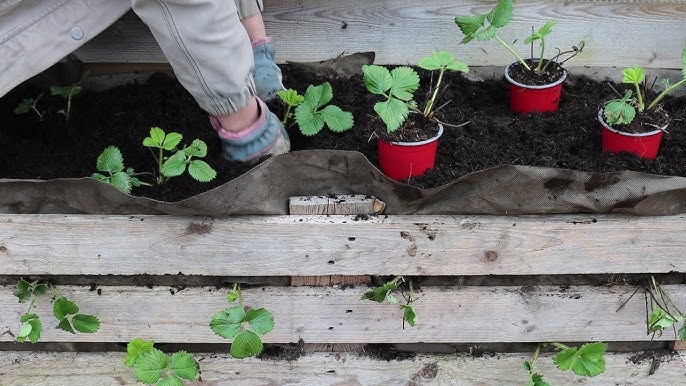In the photograph, a young woman with long, wavy blonde hair that cascades down to her waist is seen crouching by a raised wooden crate used as a planter. The setting appears to be a greenhouse, as suggested by the grooved plastic panels and wooden base forming the structure behind her. She is wearing a grayish-white sweater, blue jeans, and brown boots. The woman, who wears clear-framed glasses, looks directly at the camera with a cheerful smile. 

In the planter, which measures a few feet long and about a foot or two wide, there are young strawberry plants already sprouting through the soil and the sides of the crate. Text above the planter reads "Grow a Dozen Strawberry Plants," with emphasis on "a dozen" in yellow font, and a red arrow points toward the planter, guiding the viewer's attention. The ground around the crate is scattered with fallen leaves, adding to the detailed setting of the image.